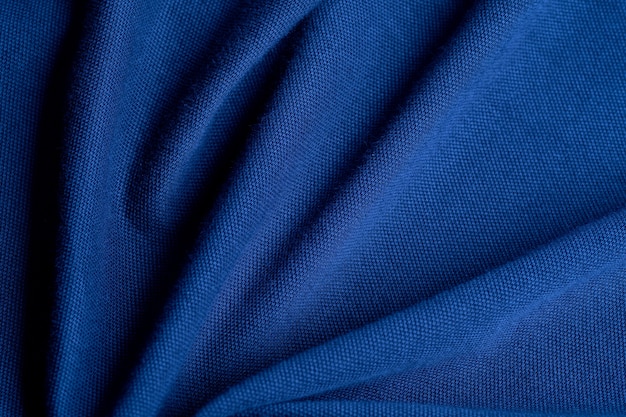This photograph captures a close-up section of a deep blue fabric, showcasing a rich and vivid hue that sits between royal blue and cerulean. The material appears thick and canvas-like, defined by a loose weave of fibers that suggest a slightly rough texture, reminiscent of twill rather than the smoothness of silk. The fabric is not laid flat; it features folds and creases that create intricate shadows, indicating the presence of a carefully positioned light source. The image, professionally shot, emphasizes the fabric's detailed stitching and weave. It is oriented longer horizontally, with shadows extending from the left edge, leading into the vertical folds that angle from left to right, accentuating the textured and densely woven nature of the material.